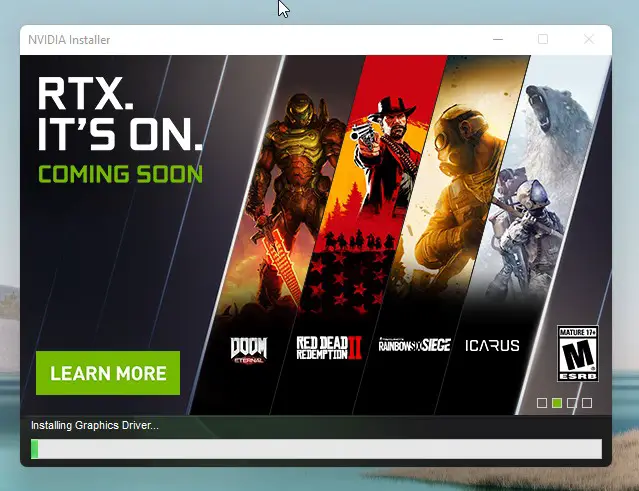In this image, we observe the process of installing NVIDIA drivers for a device. The screenshot prominently displays various game titles such as Doom Eternal, Red Dead Redemption 2, Tom Clancy's Rainbow Six Siege, and Icarus. An indication of the RTX feature being activated, alongside prompts like "Coming Soon" and "Learn More," is visible. The central focus is on the progress bar indicating the ongoing installation of the graphics driver. The image encapsulates a seamless integration of high-performance gaming visuals with advanced NVIDIA technology.